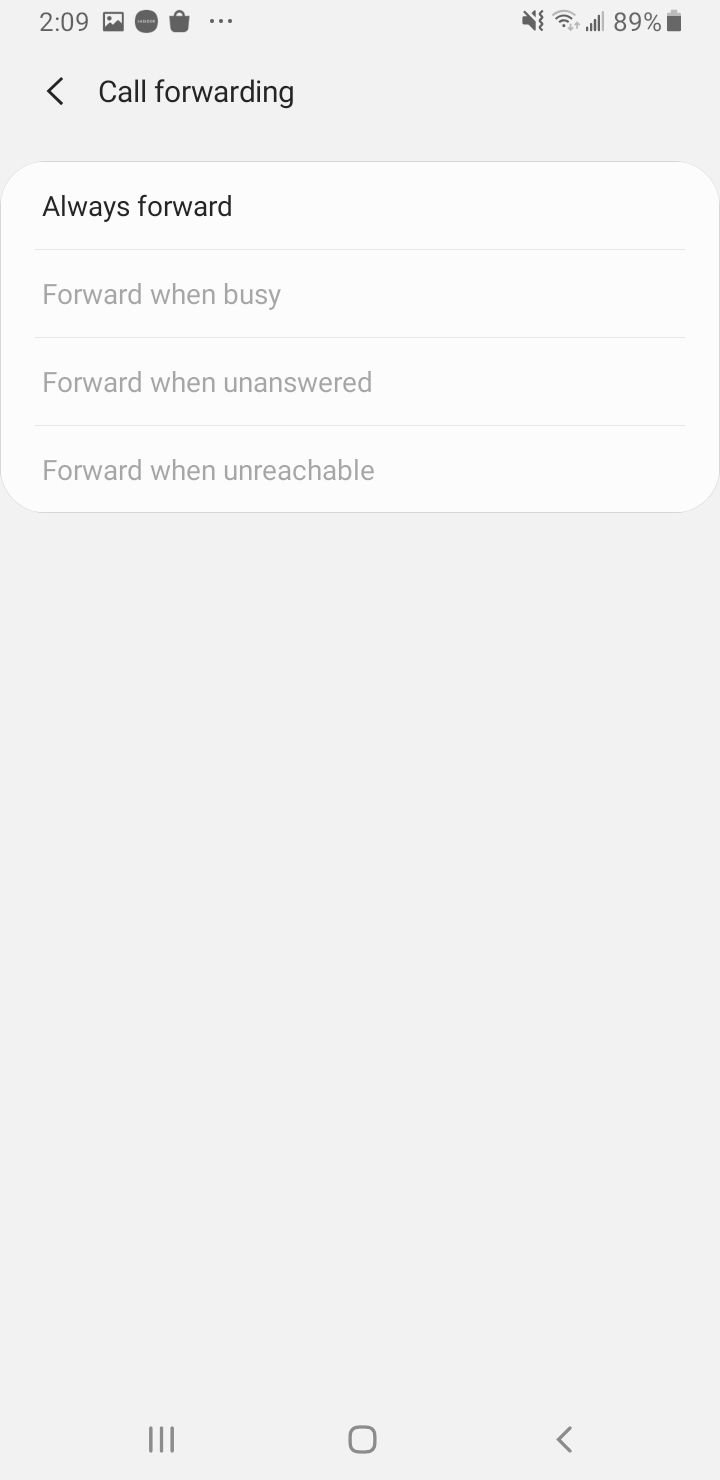The image depicts a screenshot of what appears to be a settings menu, featuring a minimalist design with a gray background and a mix of black and gray text. 

At the top of the screen, the number "209" is displayed, accompanied by an icon resembling a sun over a mountain, hinting at visual or display settings. To the right, another icon is visible, possibly indicating navigation or options, followed by a shopping bag icon and three gray dots.

On the upper right-hand side, several status icons are neatly aligned: a muted speaker icon (indicating silent mode), a Wi-Fi signal icon, a cellular signal strength icon, and a battery percentage indicating 89%.

Below this status bar, the heading "Call Forwarding" is prominently displayed in black, accompanied by a back arrow for navigation. 

The main section of the menu is enclosed in a white box divided by thin gray lines, clearly separating four options. The first option, "Always Forward," is highlighted in bold black text, while the subsequent options — "Forward when busy," "Forward when unanswered," and "Forward when unreachable" — are presented in gray, indicating potential sub-settings.

At the bottom of the screen are navigation aids comprised of three gray lines, a gray square box, and a gray back arrow, sitting above a larger, faintly outlined gray box that seems to serve as a footer or additional navigation bar.

Overall, the image is of excellent quality, crisp and clear with no pixelation or blurring, making it highly accessible and easy to interpret even for users with low vision. There are no other images or notable elements outside of what has been described.